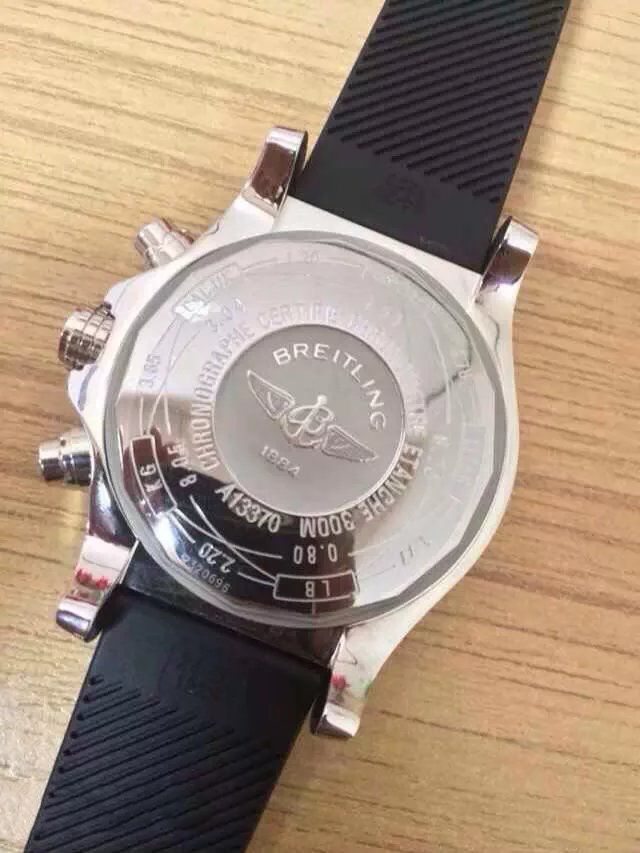This vertical, rectangular color photograph captures the back of a Breitling watch placed on a light brown wooden surface with visible darker grain lines. The watch, centered in the middle of the image, features a large, circular silver back that is very shiny. The name "BREITLING" is prominently displayed in all capital letters, and below it is the brand's logo, a schematic image resembling a letter B with wings, possibly symbolizing an eagle with outstretched wings. There's also the number "1884" inscribed below the logo, among other difficult-to-read numbers and information that might include weight measurements in pounds and kilograms. The black band of the watch, likely made of rubber or plastic, extends outward but is truncated by the photo's edges at the top right-hand corner and bottom left-hand corner. On the left side of the watch, there are three large buttons or knobs: one in the center and two situated above and below it at angles.